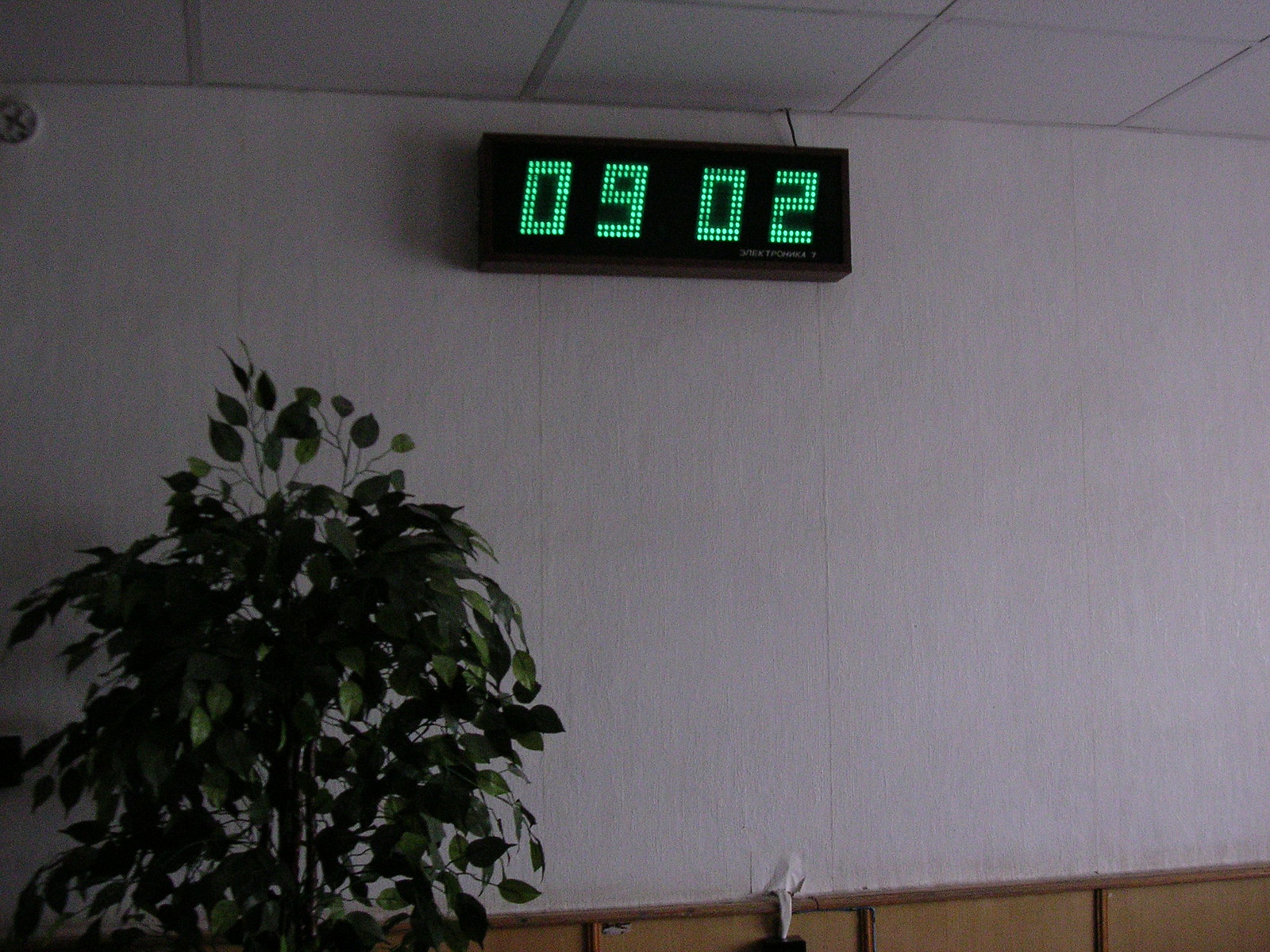The image captures a high-ceilinged space featuring a tiled ceiling. Prominently displayed on the wall is a tall, black-framed clock. Below the clock, green-lit digital numbers read "09:02:09," with the digits made of bright green lights against a dark background. The wall behind the clock is white, creating a stark contrast with the clock and numbers. The bottom section of the image shows various brown elements, suggesting furniture or architectural details in brown tones. On the left side of the image, there is a lush plant with multiple green leaves, and nestled within the foliage is a tree-like structure with rough, brown bark.